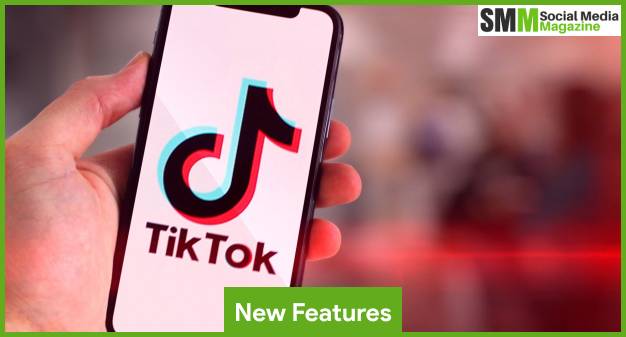This image is a screenshot of an advertisement for "SM Social Media Magazine." The entire box is dominated by an image outlined with a thin green stripe. In the top right-hand corner, the initials "SM" in black, followed by another "M" in green, signify the magazine's title. "Social Media" is in black text, while "Magazine" is highlighted in green, all set against a white background.

The main body of the image features a completely blurred background with indistinct shapes that might be people, though they are unrecognizable. In the bottom center, a green rectangle with the text "New Features" in white stands out. On the left side of the photo, a man's left hand holds a cell phone displaying the TikTok logo and the word "TikTok." The man's thumb, index, middle, and ring fingers are visible, but his pinky is obscured. A blurred red line, which might be vertical or horizontal, extends from the ring finger, adding a dynamic yet unclear element to the image. The top left-hand corner of the advertisement is a dark gray shade, providing a subtle contrast to the overall composition.